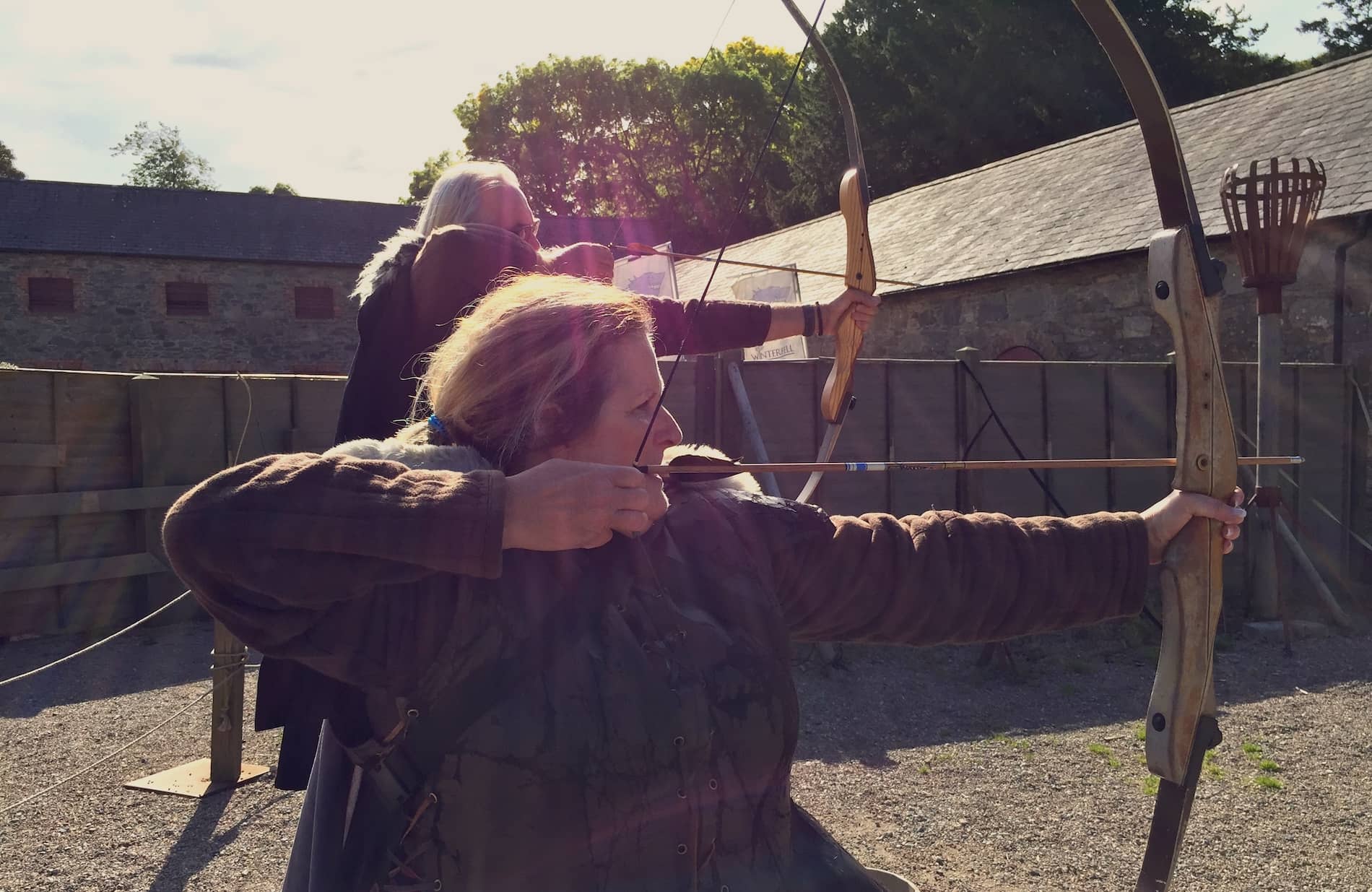In this outdoor daytime photograph, a woman and a man are practicing archery. The woman, positioned in the foreground, wears a heavy brown outfit with long sleeves and has light brown hair highlighted by the sun. She holds a recurve bow, brown in color, with its string drawn back, ready to release a wooden arrow adorned with white and blue stripes and white feathers just beneath her nose. Behind her, a man with gray hair can be seen with a similar bow and arrow, which he aims slightly downward to the left. He appears to be wearing a black t-shirt. They are both standing on a gray gravel surface with patches of green grass.

The background reveals a gray building with a steep, shingled roof to the right, and dark green trees alongside another tree with visible sky and sunlight filtering through its leaves. A metal pipe with a hollow container held by straps is also visible to the right. The sky above is light cream in color, accentuated by the bright sunlight piercing through the foliage. The overall scene is bathed in natural light, providing a clear and detailed depiction of the archery practice and the surrounding environment.